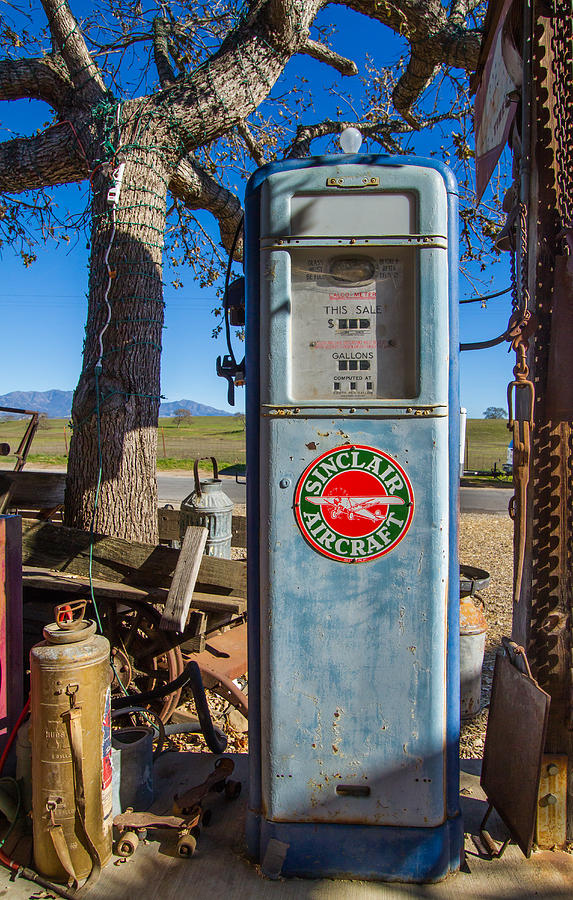In this vertical photograph, an old, rusted gas pump from potentially the 1930s to the 1960s stands at the center, slightly to the right, against a vibrant blue sky with trees adorned with Christmas lights. The gas pump, a faded light blue now marked by rust and scratches, features a prominent circular Sinclair Aircraft logo. The logo consists of a cherry-red outline, a green inner circle with "Sinclair" and "Aircraft" in white all-caps text, and a white biplane with a cherry-red outline at the center. Above the logo, a display area marked "This Sale," with spaces for three black numbers under a dollar sign, and "Gallons," similarly accompanied by empty numerical slots, indicates its analog nature. At the very top, a non-illuminated light bulb is affixed. To the left side, where the pump nozzle would typically hang, the hose is absent. Flanking the pump are various collectibles and old items, some rusted and some well-preserved, including a copper-colored tank, an old fuel tank, a flat-fronted shovel, roller skates, and a wheelbarrow filled with wood pieces. The scene takes place in a roadside area cluttered with these items, adding to the air of nostalgic decay. A road runs horizontally across the background with grassy patches and distant mountains completing the picturesque yet dilapidated setting.